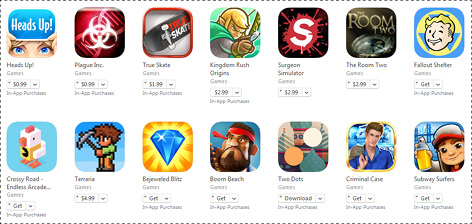This image depicts a shopping interface showcasing various in-app purchases for games and applications. The entire display is framed by a gray, dotted line forming a rectangular border. Within this rectangle, two rows are neatly organized with seven game icons each, reflective of their in-app purchase options.

In the top row, starting from left to right, the featured games include:

1. **Heads Up** - Priced at $0.99.
2. **Plague Inc.** - Priced at $0.99.
3. **True Skate** - Priced at $1.99.
4. **Kingdom Rush Origins** 
5. **Surgeon Simulator**
6. **The Room Two**
7. **Fallout Shelter**

The bottom row continues with another set of diverse game options:

1. **Crossy Road**
2. **Bejeweled Blitz**
3. … [and several other games, descriptions not fully detailed].

Each game icon is accompanied by its title and corresponding price, providing clear information about the cost associated with the in-app purchases. The structured layout and clear pricing make it easy for users to browse and select their desired app enhancements.